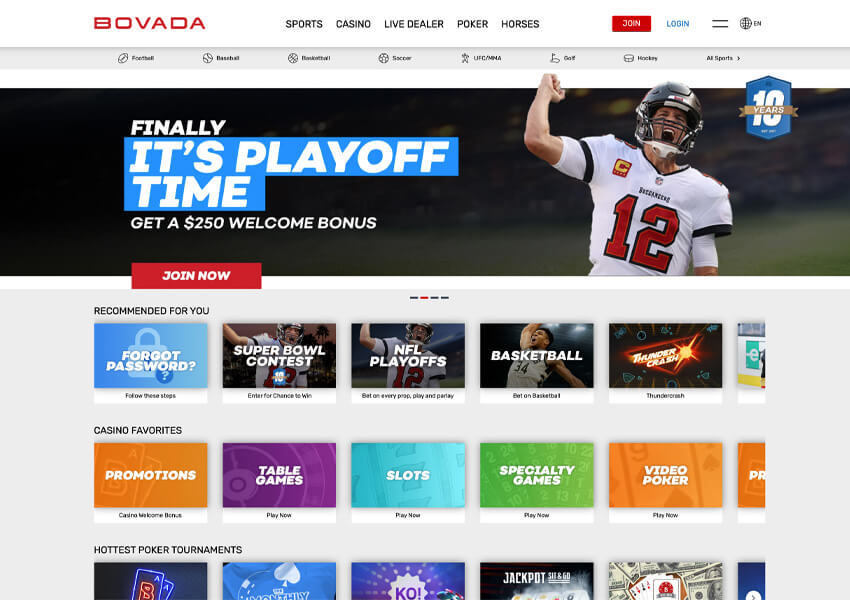The image showcases a sports betting website called Bovada, prominently displayed on the left in red. The site features five primary categories: Sports, Casino, Live Dealer, Poker, and Horses, positioned to the right of the main logo. Adjacent to these categories, there's a red "Join" button and a blue "Login" option, accompanied by a tab menu.

Beneath the main navigation, there are eight additional categories, followed by a dynamic image of Tom Brady in his Buccaneers uniform. Brady is captured from a front view, his left arm raised in the air as he appears to be shouting. To the left of Brady's image, bold blue text commands attention with the phrase "Finally, It's Playoff Time," alongside an enticing offer: "Get a $250 Welcome Bonus." 

Below this promotional banner, a large red "Join Now" button is prominently featured. The lower section of the website presents itself with three horizontal rows. The top row, labeled "For You," includes categories like "Forgot Passwords," "Super Bowl Contests," "NFL Playoffs," and "Basketball," with the fifth category being unreadable. The next row, "Casino Favorites," includes "Promotions," "Table Games," "Slots," "Specialty Games," and "Video Poker." The third row is designated as "Hottest Poker Tournaments."

The website's background is a light gray, adding a subtle contrast to the various sections and elements. Additionally, at the bottom, there are five small images of different games, further illustrating the diverse offerings of this online betting platform.